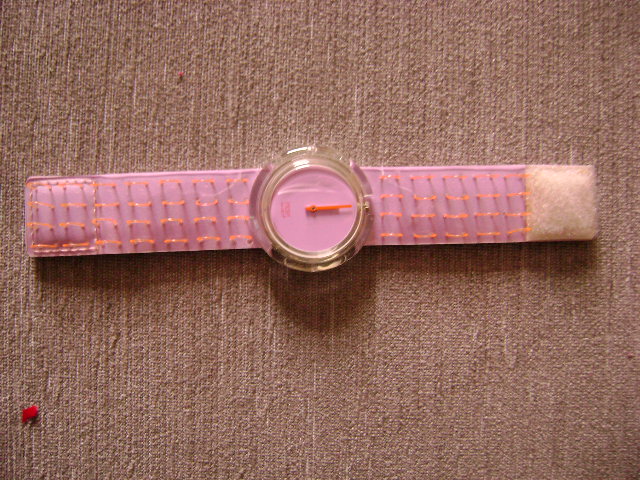The image showcases a pink watch resting on a light brown carpeted surface. The band of the watch is pink, accented by white Velcro at the end and orange stitching running along its length. The watch's face is made from clear plastic, with pink coloration and orange hands pointing to the 12 o'clock position. Distinctly, the face lacks any numerical markers. Orange details and stripes further embellish the watch. Additionally, the scene includes two pieces of red lint, one larger in the bottom left corner and a smaller one in the upper middle left quadrant. The watch and its shadow are centrally positioned within the image.